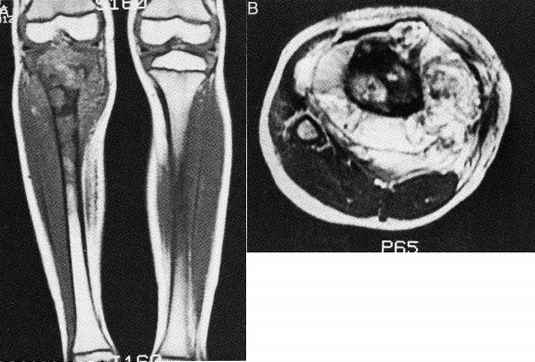The image contains two black-and-white medical radiographs. On the left, labeled as Image A, there is an x-ray showing the front view of human legs from just above the knees down to the ankles. The details of the long bones, knees, cartilage, and other tissues are clearly visible, along with some alphanumeric sequences, possibly "A12" in the top left and "S1621" in the top middle of this x-ray. On the right, labeled as Image B, there is a circular x-ray image, likely of a brain, showcasing varying shades of black and white. The image has a distinct white ring around it, with black areas transitioning to a central black circle featuring white splotches. The bottom middle of this x-ray is marked "P65."